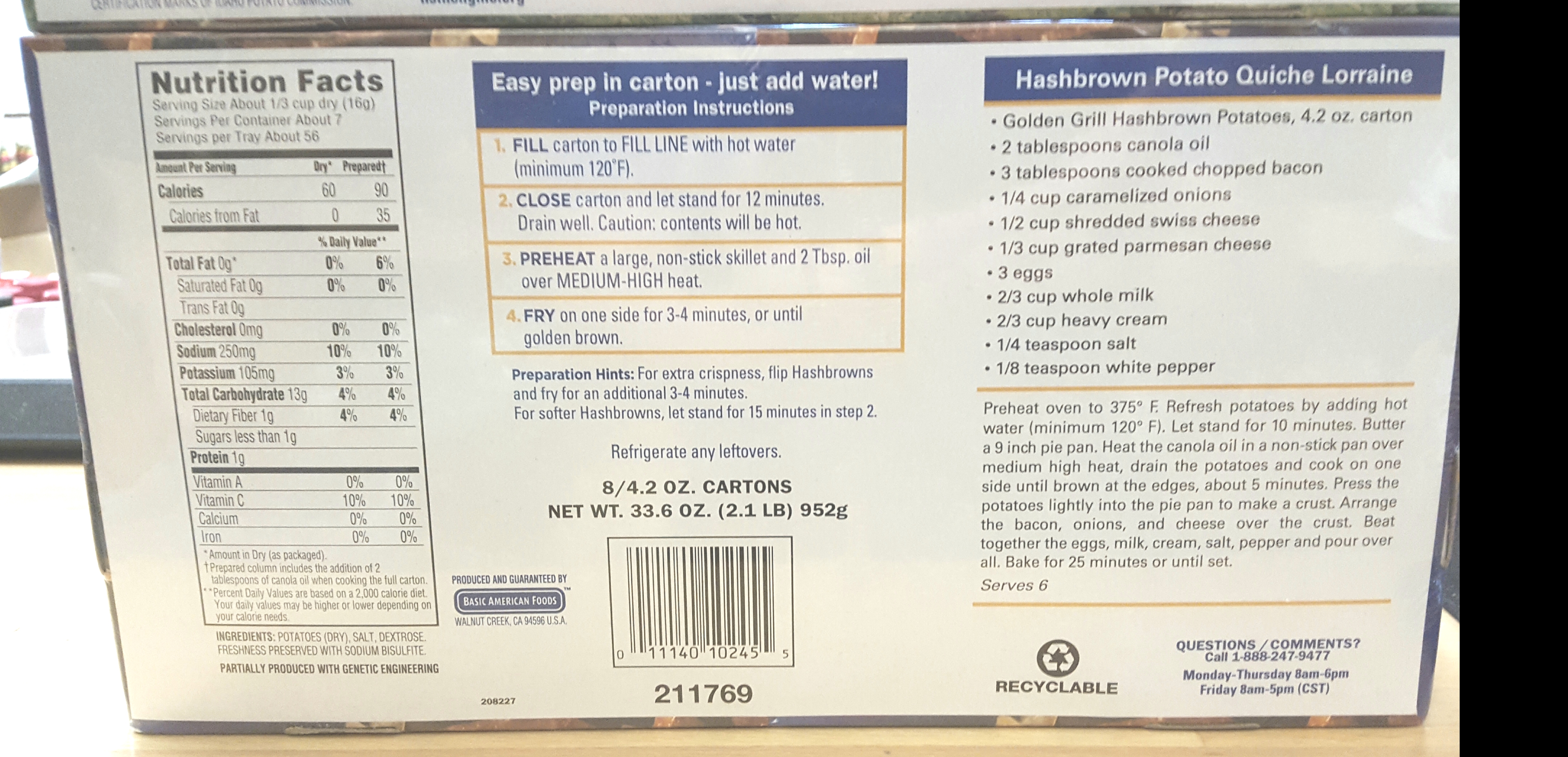The image depicts the back panel of a food product package, meticulously organized into three main sections. 

On the left side, there's a detailed nutrition facts panel outlined in black, providing key dietary information. It includes the amount of calories, fat, cholesterol, sodium, potassium, total carbohydrates, and protein present in the product. Additionally, it lists the vitamins and their corresponding daily value percentages.

The center section contains the preparation instructions labeled "Easy Prep In Carton - Just Add Water." This is followed by four detailed steps on how to prepare the food item. Below the preparation instructions, a barcode and the product's weight are displayed. 

On the right side of the panel, there's a recipe titled "Hash Brown Potato Quiche Lorraine." This section lists the necessary ingredients and provides step-by-step cooking instructions. Beneath the recipe, the recycle icon is prominently shown with the word "Recyclable" indicated underneath. In the lower right corner, there are contact details including questions, comments, and a phone number for customer support.

This detailed arrangement ensures that all essential information, from nutritional content to cooking instructions, is easily accessible to the consumer.